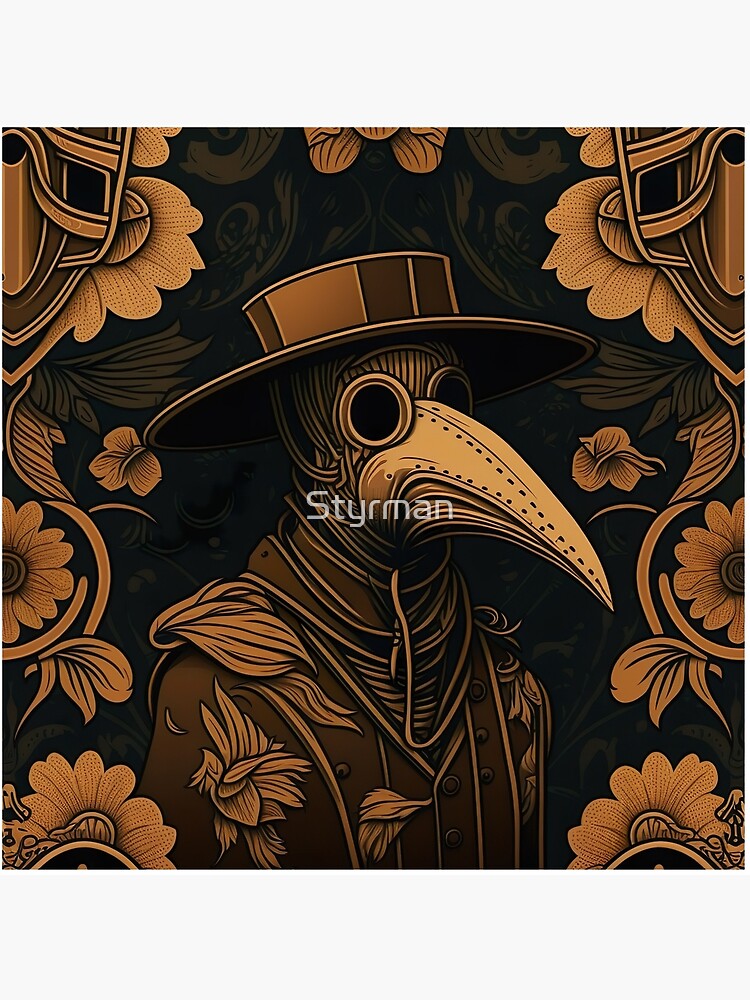This is a detailed digital illustration depicting a mysterious humanoid figure adorned in elaborate attire. The background is a dark gray with intricate decorative elements in copperish and goldish hues, representing foliage, flowers, vines, and ribbons, appearing as though they are hammered into leather. The central figure, which stands three-quarters to the right and appears from the chest up, resembles a bird dressed in human clothes, creating a unique caricature.

The figure wears a large, flat-brimmed hat in a brown and gold color palette that snugly fits the head. Covering the face is a mask with large, black, goggle-like eyes and a long, stitched, orange beak protruding forward. Wrapped around the figure’s head are string-like elements. The ornate jacket features a three-piece suit design embellished with floral patterns and tassel-like designs hanging from the shoulders. The entire image, contained within a perfectly square frame, exudes a sense of timeless artisan craftsmanship combined with digital artistry, creating a striking piece that merges human and avian elements in a beautifully detailed composition.